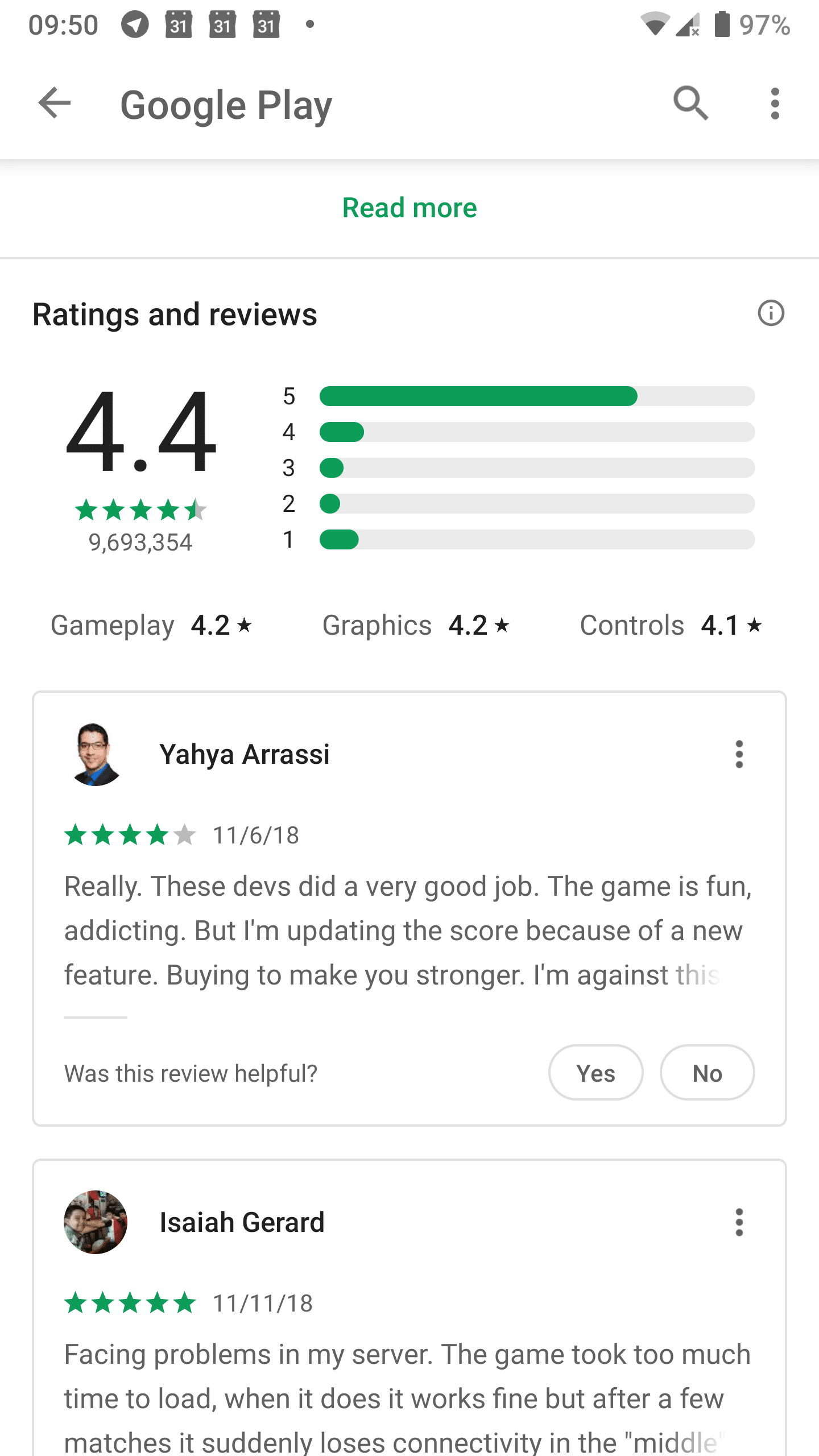**Detailed Descriptive Caption:**

This color portrait-format screenshot captures a smartphone screen at 9:50 AM with the battery life displayed at 97% and medium connectivity reception. The top of the screen is cluttered with various icons, including the calendar app, indicating background activity. The currently open app is Google Play, where the user has scrolled down slightly on a specific app’s page. The partially visible content begins with a "Read More" link. Below this, the app boasts a rating of 4.4 stars from approximately 9.7 million reviews. Detailed ratings include 4.2 for Gameplay, 4.2 for Graphics, and 4.1 for Controls, hinting that this could be a gaming app. The page also displays user reviews with dates from 2018.